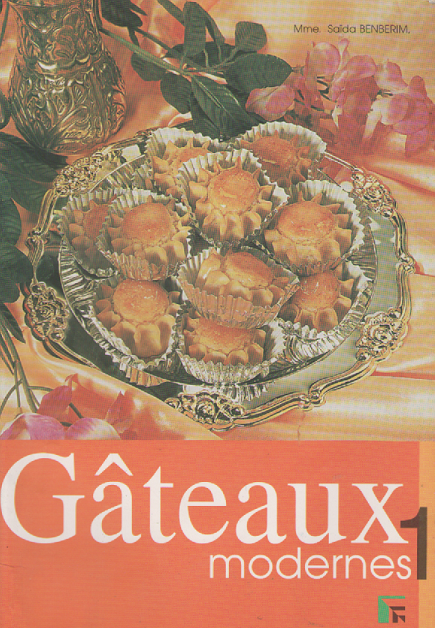The image is likely the front cover of a magazine or cookbook. It features a beautifully ornate silver plate at its center, holding a selection of circular pastries. Each pastry, housed in a muffin cup, has a sun-like design with a filling in the middle, reminiscent of cookies or muffins. Surrounding this central plate on either side are pink flowers with green leaves, adding a touch of natural elegance to the scene. To the upper left corner, there is a partial view of a silver pitcher or candlestick.

The backdrop of the image consists of a table adorned with a goldish-yellow tablecloth, creating a complementary contrast with the pink and peach tones of the flowers and overall background. The bottom third of the image contains text in French, written in white on an orange background. The text reads "GATEAUX MODERNES," followed by the number "one" in brown lettering, suggesting a thematic focus or perhaps indicating a volume number. Overall, the composition hints at a sophisticated presentation, likely related to baking or elegant desserts.